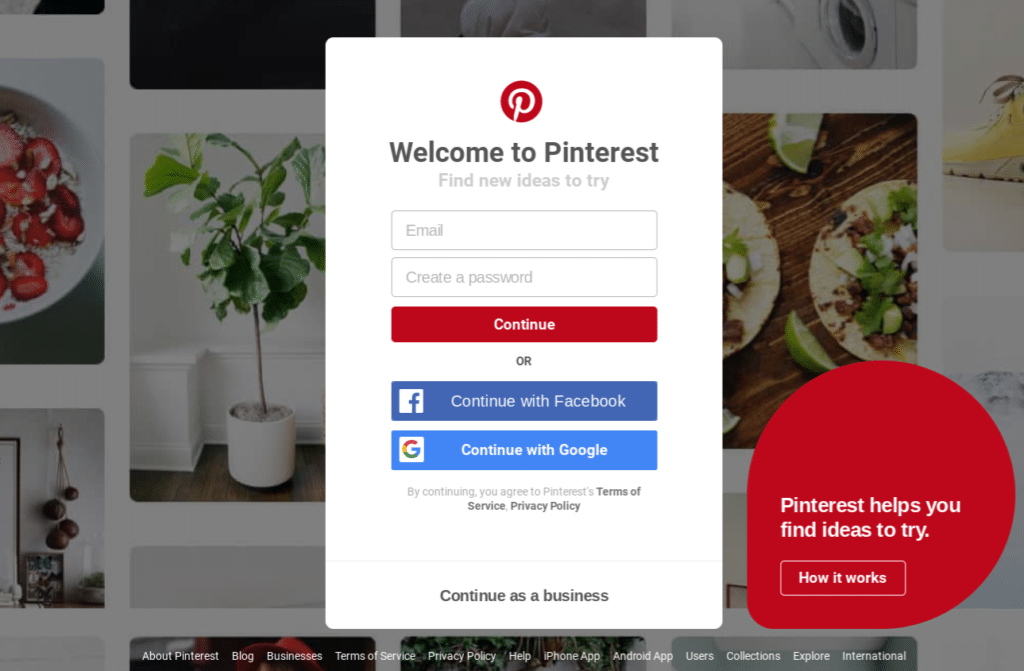Screenshot of the Pinterest Website:

The screenshot captures the Pinterest homepage with an overlaying white pop-up window in the center. The background consists of a mosaic of grayed-out images due to the overlay effect. Visible images include a white bowl filled with a red food item, a plant in a white pot, tortillas, and pieces of furniture.

The pop-up window features the Pinterest logo at the top—a red circle with a white stylized "P" in the center. Beneath the logo, it reads: "Welcome to Pinterest. Find new ideas to try." Below this prompt, there are fields and options for user interaction: "Email, create a password," along with buttons to "Continue" or "Continue with Facebook," and "Continue with Google." It also notes that by continuing, users agree to Pinterest's Terms of Service and Privacy Policy, with an additional option to "Continue as a business."

In the bottom-right corner of the screenshot, there is a red teardrop-shaped icon with text stating, "Pinterest helps you find ideas to try." Following this, "How it works" is displayed.

At the very bottom of the screenshot, a footer lists various Pinterest-related links and resources: "about Pinterest, blog, businesses, Terms of Service, Privacy Policy, help, iPhone app, Android app, users, collections, explore, international."

The image does not contain any people or animals.